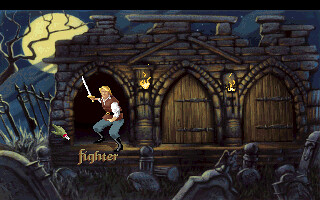The image appears to be a nighttime screenshot from a medieval-themed video game. The sky is a dark blue, almost black, and a bright yellow moon illuminates the scene. On the left side of the image, there's a bare tree with no leaves, and below it, what appears to be headstones or crosses indicating graves.

Dominating the scene is a person identified as a "fighter." This individual is depicted waving a silver or white sword. He is dressed in a white shirt with a brown vest, gray or blue pants, black boots, and something on his head akin to a pirate's headgear. Below him, the word "Fighter" is displayed in yellow text.

The fighter stands before a large stone building that features three brown wooden doors. This building is partly illuminated by torches affixed outside the doors, casting a fiery glow on the surroundings. At the bottom right and center of the image, there appear to be stone objects or statues scattered around. The fighter seems poised for action, possibly addressing a crowd or preparing for a confrontation.